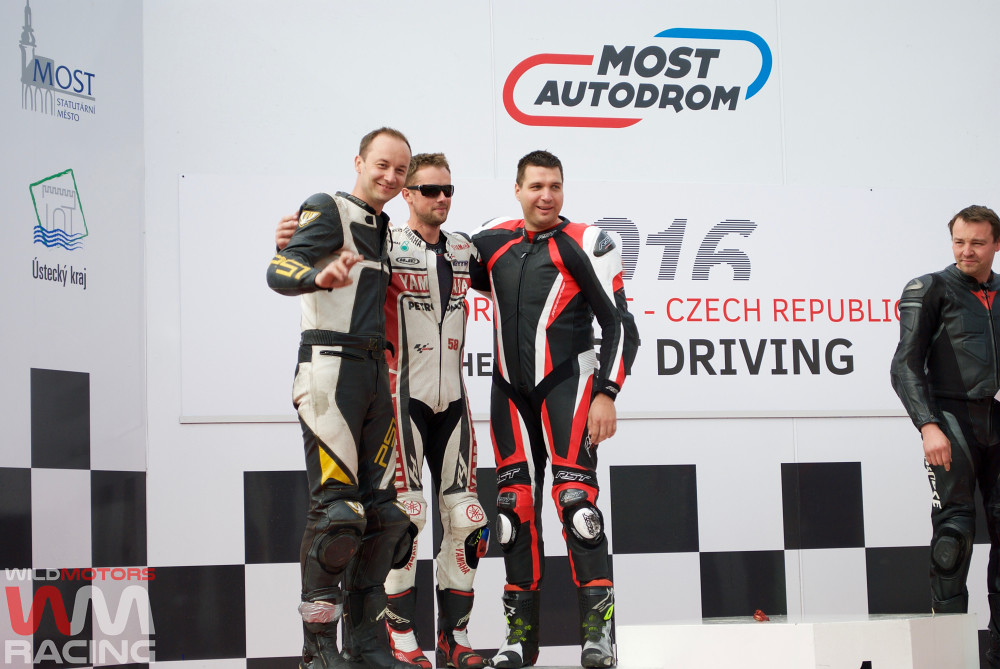The image shows four men in distinctive automotive racing uniforms standing on a podium stage. The men are posed in front of a backdrop, which features a prominent black and white checkered pattern typically associated with car racing events. In the background, text on the white wall reads "Mos Audrum" and includes references to the Czech Republic, suggesting the event's location. From left to right, the men are wearing jumpsuits in various color schemes: one in all white with black trim, one in black with red and white trim, and one in white and red. The tallest man stands on the left, while the middle man, who wears dark sunglasses, and the rightmost man are of similar height. The fourth man, standing slightly apart to the right and slightly turned towards them, also wears a black racing suit. The podium and uniforms hint that they likely just finished participating in a race. The image includes a watermark in the bottom left corner that reads "World Motors WM Racing" in red and white text. The scene appears to be captured in daylight, given the brightness, and there are no visible spectators in the background.